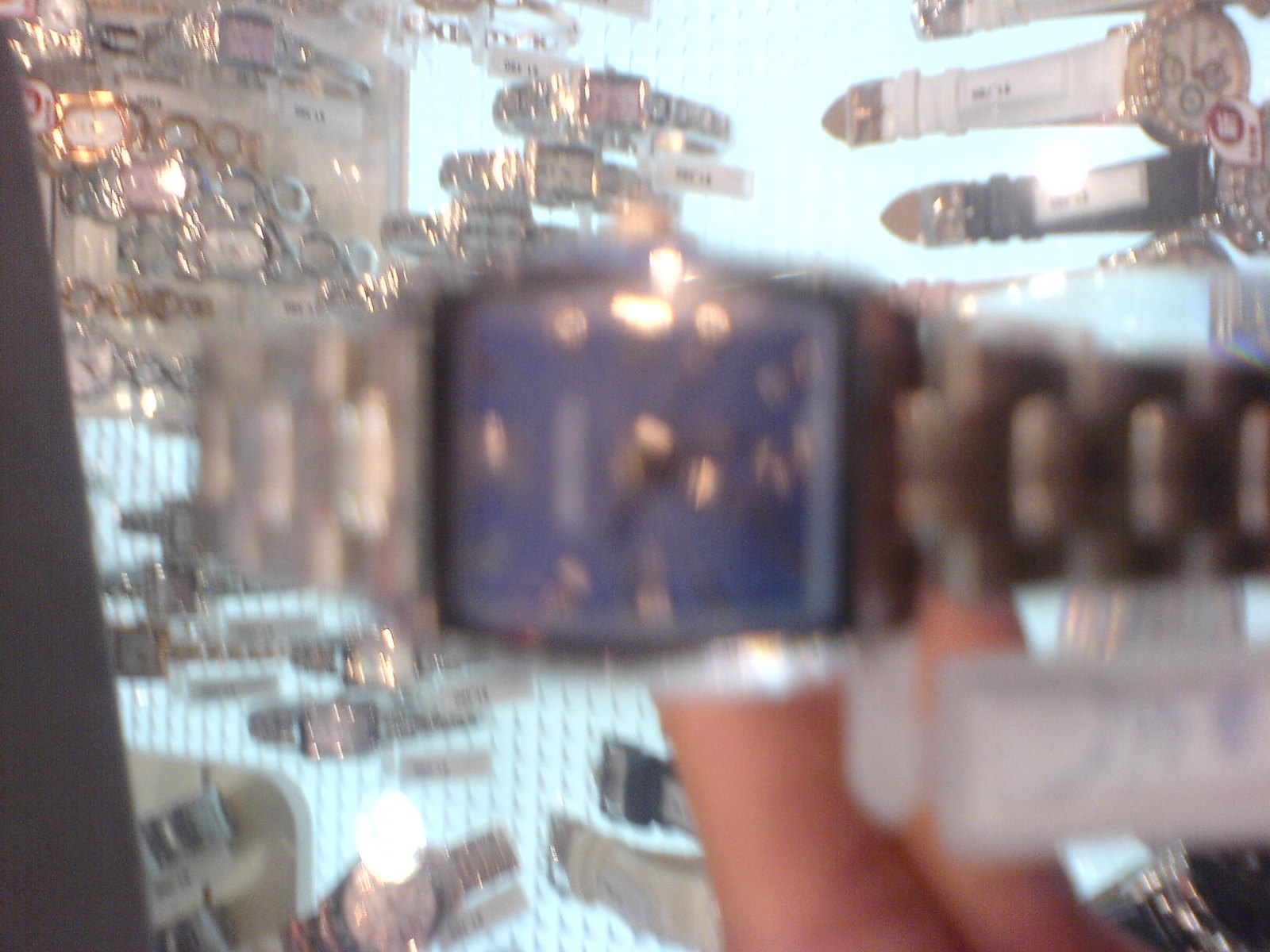The image is a realistic, horizontal rectangular photograph taken inside a watch store, showcasing a diverse display of watches. The central focus of the photo is a man's watch, which is being held up close to the camera by a person with light skin. This watch features a stainless steel or silver wrist strap and a blue face, though the numbers and hands are blurry. Attached to the watch is a white price tag with blue lettering, also out of focus.

In the background, the display includes approximately 50 watches with metal frames and straps, arranged in various rows and columns. These watches come in different colors including metallic, gold, black, and white. They appear to be organized on transparent shelves that create an illusion of the watches floating in the air. The entire backdrop resembles a light blue or white pegboard, adding to the overall store display aesthetic. The photograph is slightly blurry with glare from the reflective surfaces of the watches, contributing to the overall hazy appearance of the scene.